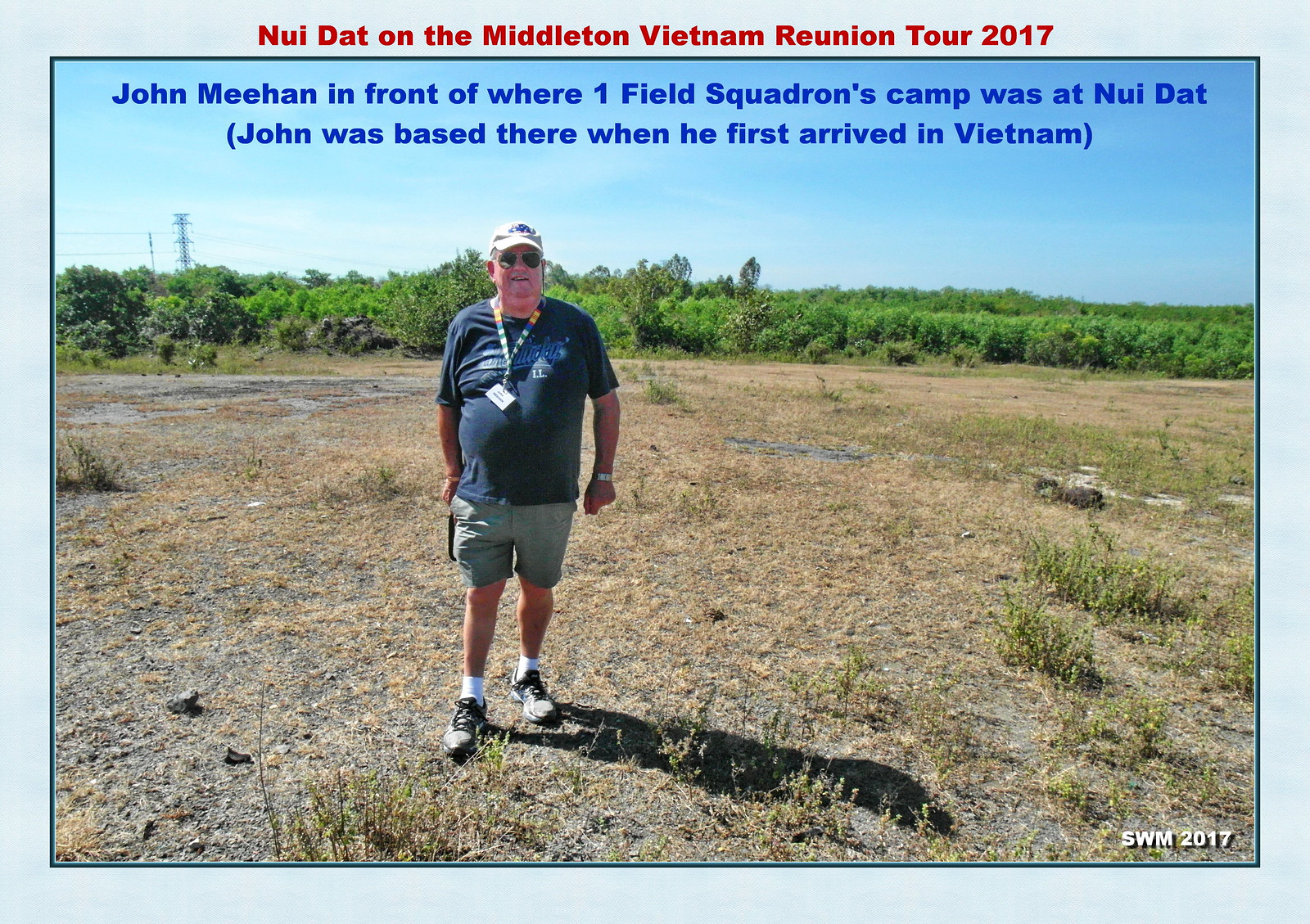The photograph, taken on a bright day outside, features an elderly white man standing in a dry, flat terrain with dirt, patches of dead grass, tall green weeds, and scattered dry brush. The landscape behind him shows thick green bushes and some short trees, with power lines faintly visible in the background. The man, identified as John Meehan, is smiling at the camera. He is dressed in a white cap, aviator glasses, a blue short-sleeve shirt, gray shorts, black shoes, and white socks, with a lanyard hanging from his neck. Above him in blue text, it reads: "John Meehan in front of where 1 Field Squadron's camp was at Nui Dat," and further notes, "John was based there when he first arrived in Vietnam." At the top of the photograph, in red font, it says: "Nui Dat on the Middleton Vietnam Reunion Tour 2017," and the bottom right corner has "SWM 2017" in white font. The image is framed by a green border, which is itself surrounded by a wide blue border.